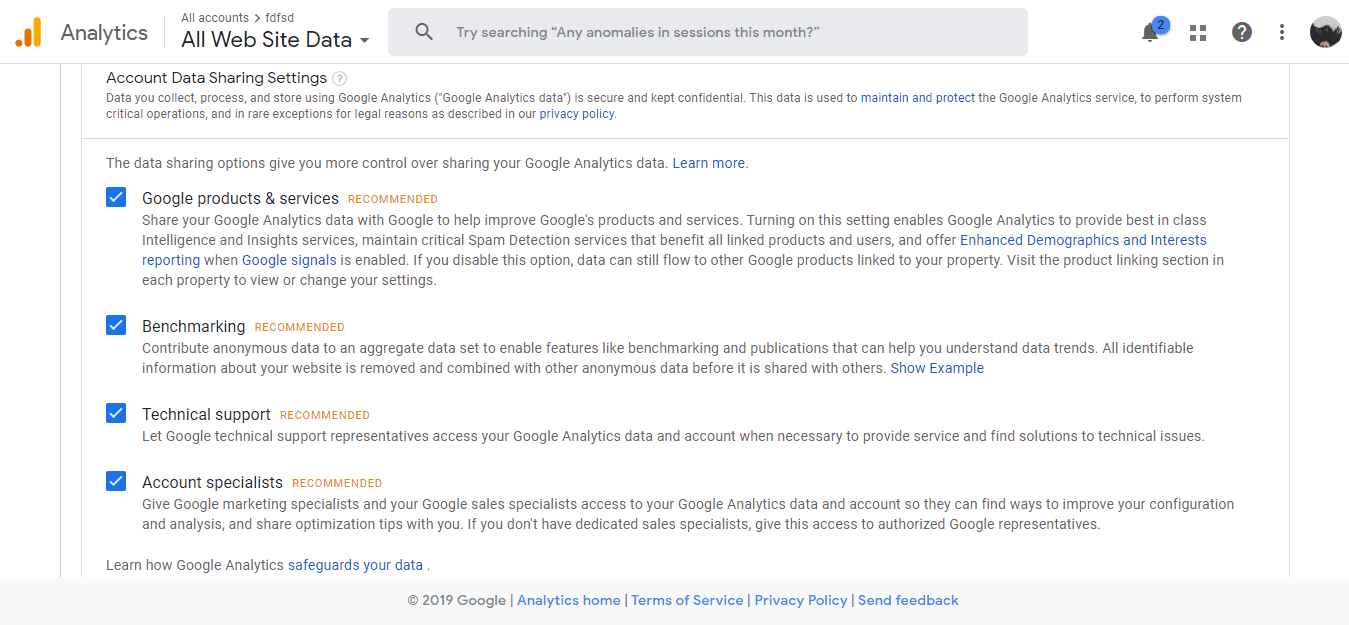**Detailed Caption:**

In the image, Google Analytics settings are displayed with various options for data sharing and user management. Users are prompted not to restrict their data usage and are encouraged to enable orange analytics for all accounts to Full Data (FD) and Full System Data (FSD). The screenshot illustrates website data settings and highlights tools like anomaly detection in sessions.

A prompt asks about the blue circles, which suggest activating account data sharing and understanding how collected data is processed and stored securely in Google Analytics. The analytics data is used to maintain and enhance the Google Analytics service, ensuring optimal performance through critical system functions.

There's an emphasis on data sharing options, giving users more control over how their data is handled and shared within the Google ecosystem. This includes enabling settings that allow for benchmarking and better utilization of Google products and services. The recommendation to turn on the setting is highlighted in orange, suggesting it benefits the service's intelligence and spam detection features.

Users are informed that enabling these settings help maintain system integrity and offers enhanced demographic reporting when Google Signals is enabled. They are also advised on how to manage data flowing to other Google products linked to their property by visiting the product linking section.

The image recommends contributing anonymous data to an aggregate dataset. This enables features like benchmarking and publications, helping users understand data trends. It reassures users that their website information is anonymized and aggregated before being shared.